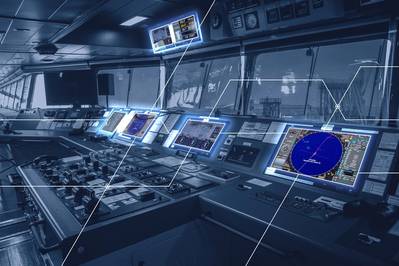The image depicts an interior shot of a control center, potentially for a ship, given the presence of radar and navigational displays. The dimly lit room features multiple monitors and panels, including three primary screens in front of large glass window panes that offer a view to the outside. The right-most monitor prominently displays a large blue circle with intricate white lines, likely representing radar information. An additional monitor is situated above the three main screens and the window panes. To the left of the center console, numerous switches and buttons are visible, suggesting a complex array of controls. The center console also houses a significant switchboard with numerous keys. Despite the absence of people, the room is brightly illuminated by daylight filtering through, revealing other details like clocks on the wall and darkened computer screens. Overall, the diverse equipment and control panels indicate this is a sophisticated operational hub, possibly a ship’s control room or another high-stakes environment such as an airline or TV studio control room.